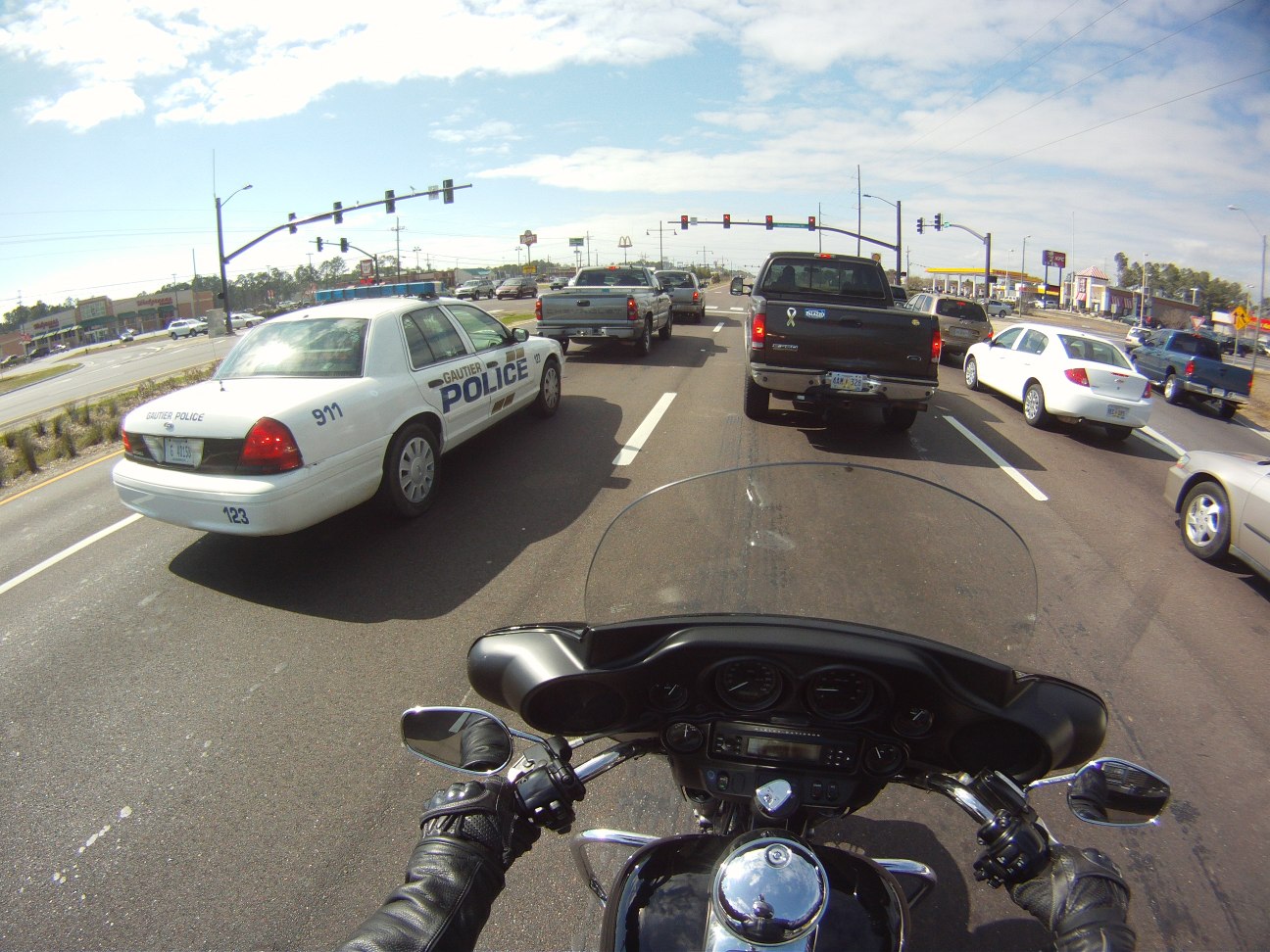The image is a full-color, point of view photograph taken from a motorcycle on a grey asphalt road with three lanes of traffic, delineated by dotted white lines and bordered by a solid white line on the side, followed by more asphalt and a solid yellow line. The sky above is light blue with multiple white clouds. The motorcycle, black with chrome trim, is shown from the rider's perspective, who is wearing black leather gloves and a black jacket with both hands on the black handlebars.

To the left, there is a white police car labeled "Gaudier Police 9-1-1" in blue text. In front of the motorcycle are several stopped vehicles at a red light, including a black pickup truck directly ahead, adorned with a yellow breast cancer awareness ribbon. The scene includes various vehicles in different colors, such as whites, blues, reds, greens, and blacks. Scattered around are buildings in yellow, red, and tan tones.

The upper right of the image features a KFC and a Shell gas station, while the middle to the right showcases more gas stations and restaurants, contrasted by a Walgreens on the left. The photograph captures the detailed reality of a typical street scene from the vantage point of a motorcyclist, stopped at a traffic light in a bustling area.